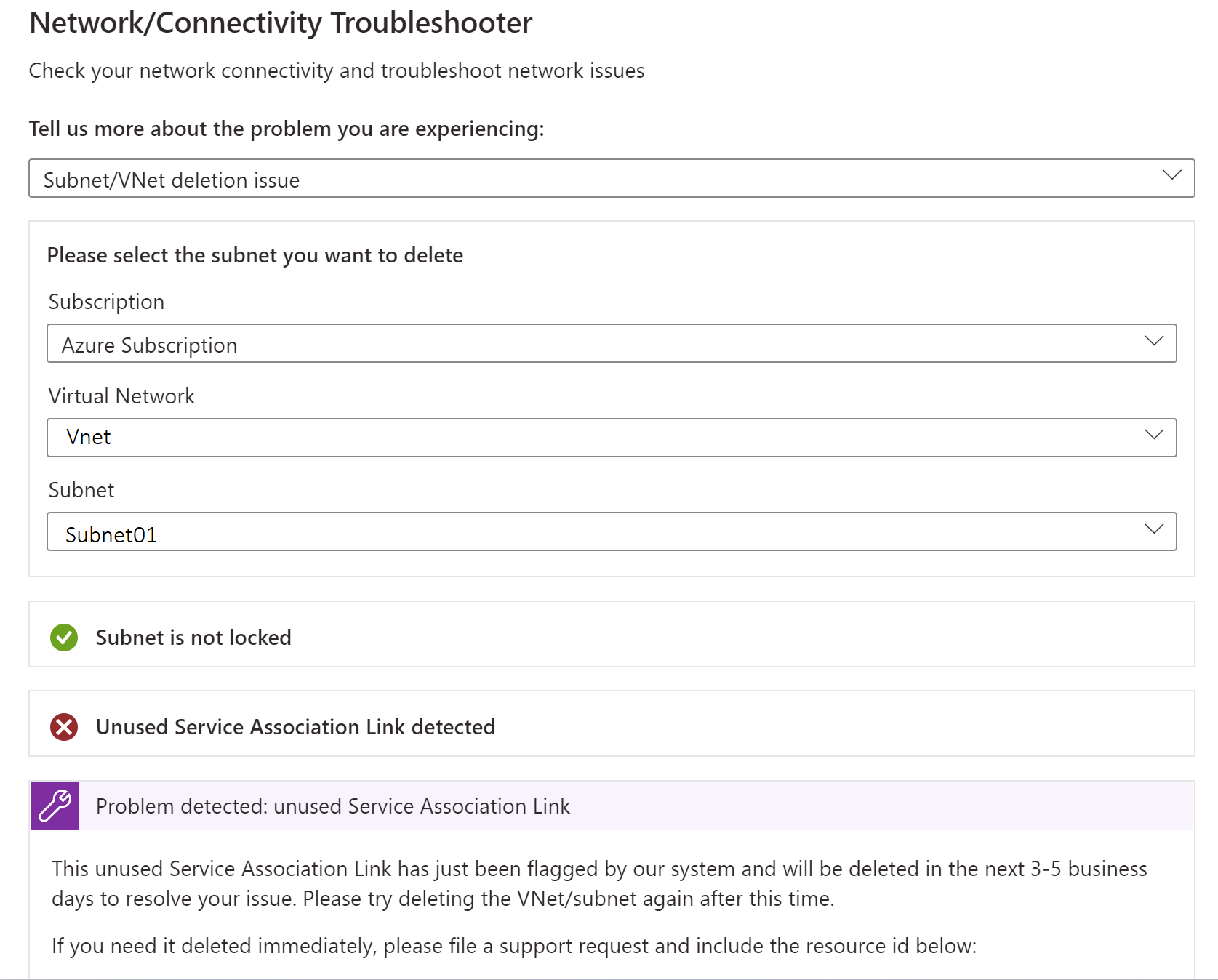**Caption:**

This image appears to be a screenshot from a web page dedicated to troubleshooting network issues on a computer. The page features a clean, white backdrop with all text displayed in black for easy readability.

In the upper left-hand corner, bold text reads "Network / Connectivity Troubleshooter." Beneath this header is the instruction: "Check your network connectivity and troubleshoot network issues." 

Following this, there is a prompt: "Tell us more about the problem you are experiencing." Below this prompt is a white drop-down tab featuring the text "Subnet / VNet deletion issue" in black, accompanied by a drop-down arrow on the right-hand side.

Further down, a section box starts with the instruction: "Please select the subnet you want to delete." The first field within this box is labeled "Subscription," containing a bar labeled "ZUR Subscription" with a drop-down arrow to the right of it. 

The next field is labeled "Virtual Network," featuring a box with the text "VNet" and an adjacent drop-down arrow. This is followed by the "Subnet" field, which contains a bar labeled "Subnet 01" in black text.

Below these fields, there is a thin box that spans the width of the page, containing a green circle with a white checkmark on the left and the text "Subnet is not locked" in black.

Underneath this section, there's a separate white box with a red circle and a white X in the left-hand corner. Next to the icon is the warning: "Unused Service Association Link Detected."

Further down, another box bears a small purple icon of a wrench in its upper left-hand corner, next to which it states: "Problem Detected, Unused Service Association Link."

The text beneath this message explains: "This Unused Service Association Link has just been flagged by your system and will be deleted in the next three to five business days. To resolve your issue, please try deleting the VNet / subnets again after this time period." 

At the very bottom, there is a note: "If you need it deleted immediately, please file a support request and include the resource ID below."